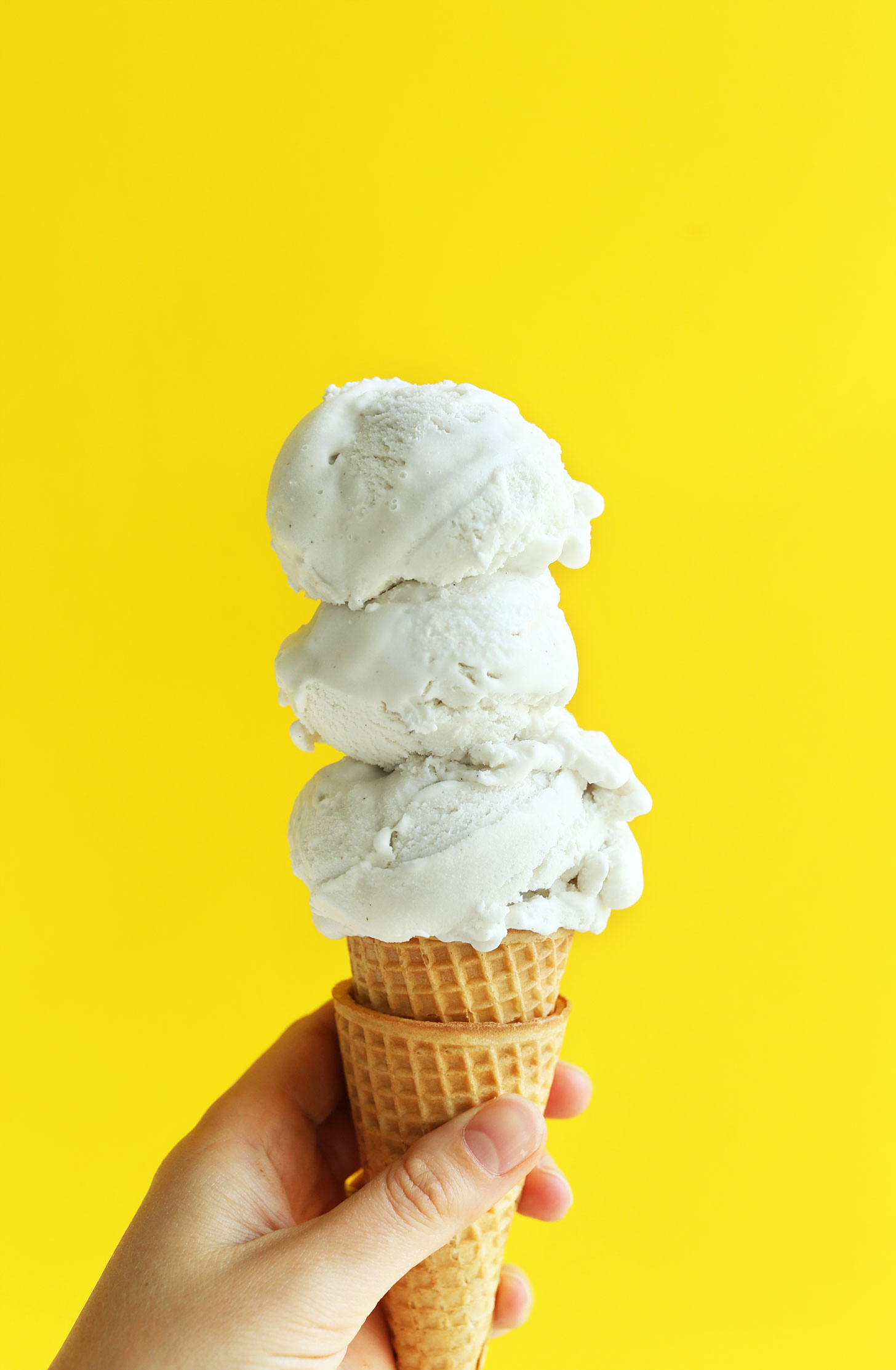In this vibrant photograph, a left hand with white skin, appearing to belong to a woman or youngster, emerges from the bottom left corner, delicately clutching a unique double-layered waffle cone. The partial view of the hand prominently displays the thumb in the foreground, while the fingers wrap around the cone's back. The cone itself is a light beige, golden brown hue, featuring a second cone nestled inside. Atop this intricate cone structure, three substantial scoops of milky white ice cream, likely vanilla, are precariously stacked. The scoops, pressed together to maintain their stability, vary in size with the largest sitting encased in the top cone, and each subsequent scoop slightly smaller and overlapping the previous. The entire scene is set against a striking, solid yellow background, creating a vivid, sunshiny backdrop for this delightful frozen treat.